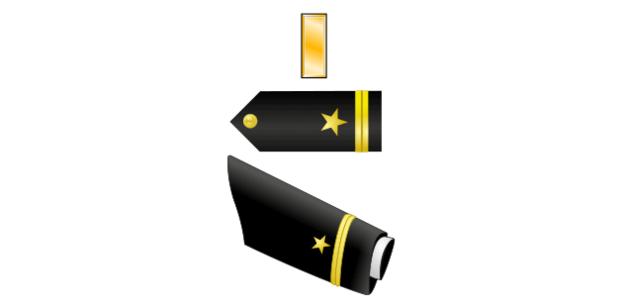The image depicts three objects presented vertically on a completely white background, resembling clip art rather than a photograph. The top object is an upright, light orange (or gold-colored) rectangular box. Beneath it are two black, tubular shapes, both featuring gold stars and stripes. The first tubular shape closely resembles an officer's insignia or the epaulet of a uniform with a distinct black form, containing a yellow star near the bottom and two yellow stripes. Its end is folded into a triangular shape. Below this is a similar black tubular shape, also adorned with a yellow star and stripes, yet slightly longer and more oblong, displaying an interior cross section or wound material as if indicating the structure beneath its surface.